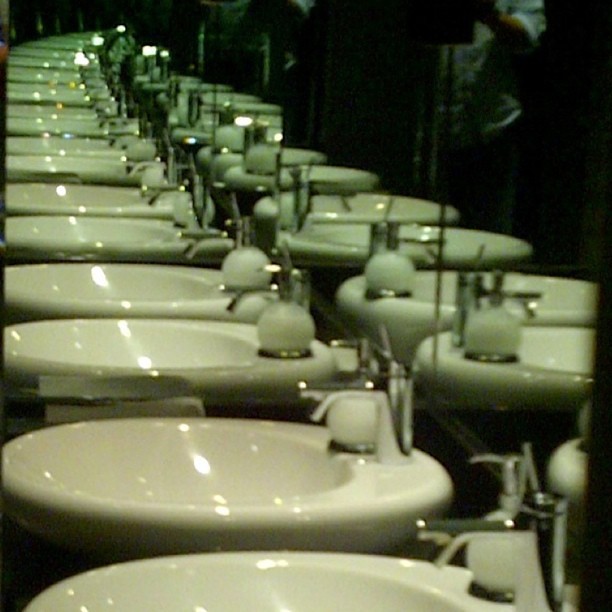The photograph captures a series of sleek, white porcelain sinks arranged in a continuous row, stretching from the foreground into the background. These sinks, which are slightly oval and shallow, are installed along a wall that bends slightly to the right, creating a mild curve in their arrangement. Each sink is equipped with modern silver faucets and a built-in, white globe-shaped soap dispenser that ascends into a cylindrical form, containing what appears to be a white liquid. The entire setup is backed by a long mirror divided into separate panes, reflecting the sinks and creating a visually infinite effect. This mirror also reveals a partial reflection of the photographer, who is wearing a floral print shirt and blue jeans. The photograph is tinged with a greenish light, adding to the surreal and stretched perspective of the sink row, which seems to extend endlessly. The ambiance and arrangement suggest that this could be a public restroom in a large gathering place.